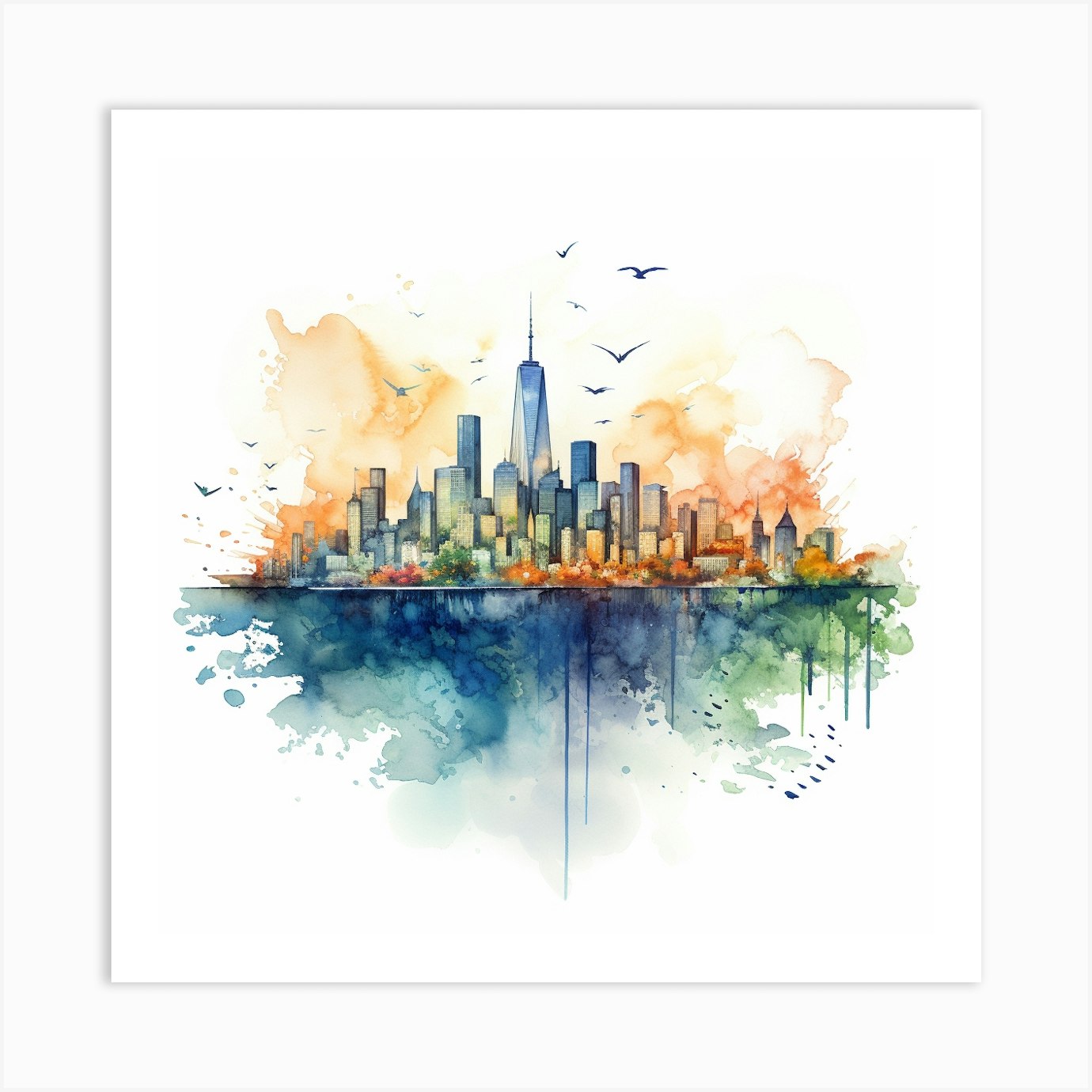This artistic watercolor painting beautifully captures a vibrant city skyline that is right on the edge of a water body, giving an impression of it being either Dubai, New York, or Chicago. The cityscape, dominated by towering skyscrapers, includes one notably tall and recognizable building centrally positioned, possibly reminiscent of Dubai’s architecture, the Chrysler Building in Chicago, or New York's One World Trade Center. The buildings are painted in a mix of bluish-green hues with hints of orange at the base, exhibiting a dynamic interplay of colors. Above the skyline, the sky features splashes of orange, evocative of sunset clouds, which blend seamlessly into the background. Below the buildings, the paint appears to drip downwards, suggesting an underground or water reflection effect, highlighted with blue and green tones. The foreground includes fall-colored foliage interspersed with green vegetation along the water's edge. Numerous birds, resembling seagulls, are depicted flying around the skyline and over the water, adding a sense of movement and liveliness to the scene.